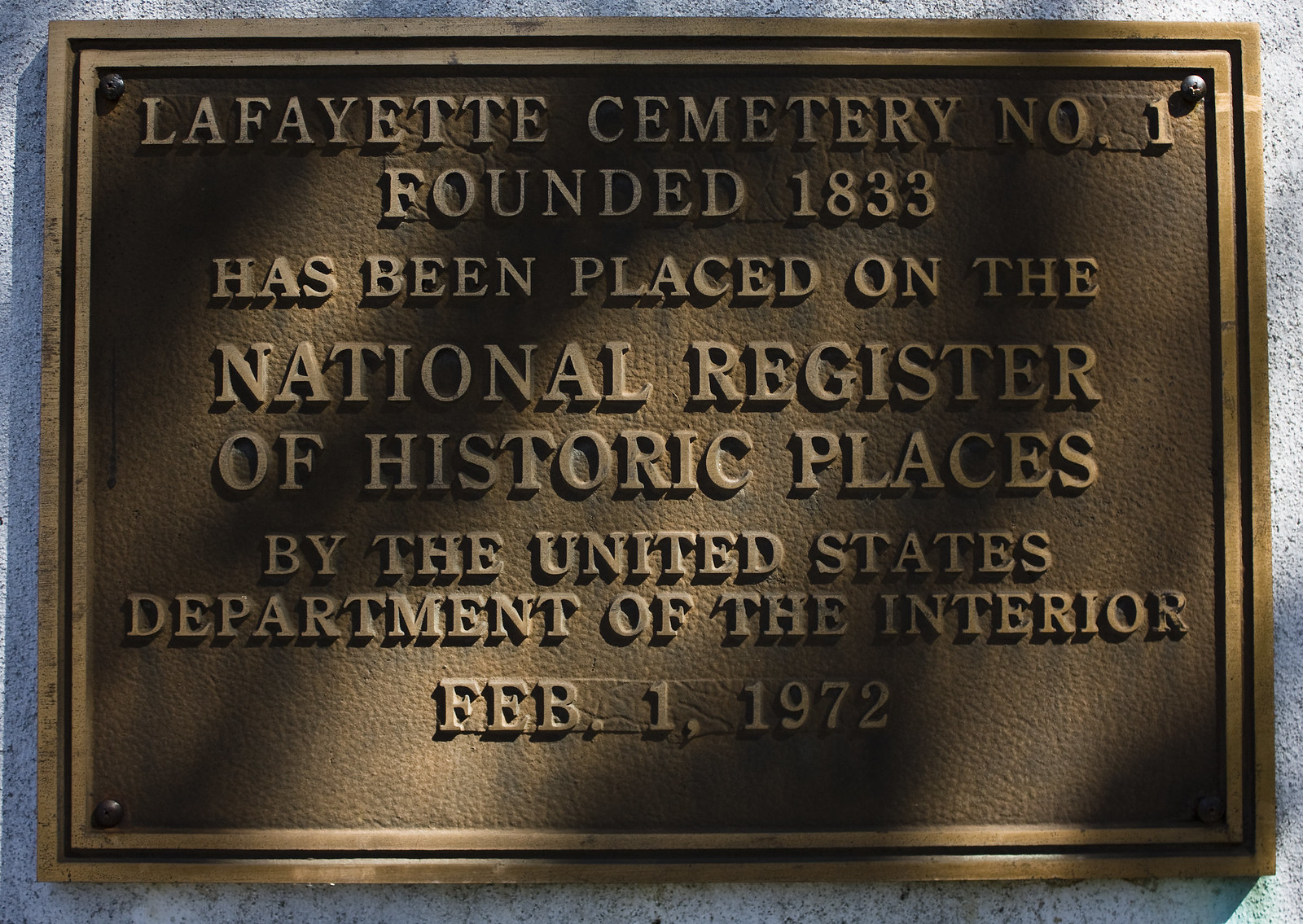This is a detailed photograph capturing a metal placard attached to a grey granite stone wall with four black screws, one at each corner. The placard features a solid bronze border framing a central leathery brown surface that is slightly aged and has raised letters. The text on the placard reads: "Lafayette Cemetery No. 1, founded 1833, has been placed on the National Register of Historic Places by the United States Department of the Interior, February 1, 1972." Despite its age, the placard shows signs of weathering and hints of rust, while the screws remain rust-free and black. The scene is bathed in sunlight, casting varied light and shadows across the plaque, indicating the presence of nearby trees or other structures catching the sunlight. Overall, the placard remains in relatively good condition, with weathered areas appearing intentional rather than extensively rusted.